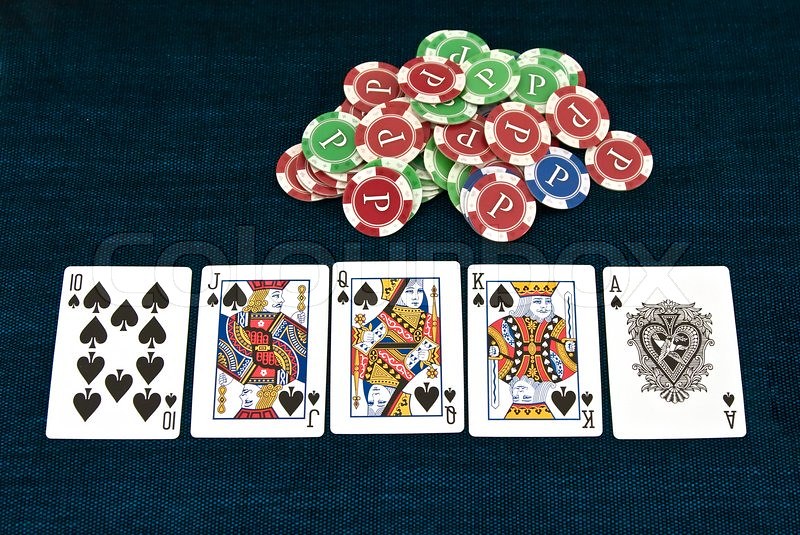The photograph features a neatly arranged display of playing cards and poker chips set against a black cloth backdrop. The playing cards, all of the spade suit, are carefully spread out in a straight line along the lower section of the image, displaying a straight flush comprising the 10, Jack, Queen, King, and Ace. Each card is aligned perfectly next to the others, creating a clean and organized visual effect.

Above this line of playing cards, there is a scattered pile of colorful poker chips. Each chip prominently features the letter "P" at its center. The poker chips come in various color combinations: red with white, green with white, and blue with white. In terms of design, the chips have intricate patterns resembling a wheel or star around the outer edge, created with alternating dashed or dotted lines in their respective colors.

The photograph also displays a faint watermark that reads "color box" (or possibly "cloud box") across the image, indicating that it is likely protected by some form of copyright or usage rights. This watermark is partially transparent and does not heavily obstruct the view of the cards and chips, allowing the details and vibrant colors to remain the primary focus of the photograph.